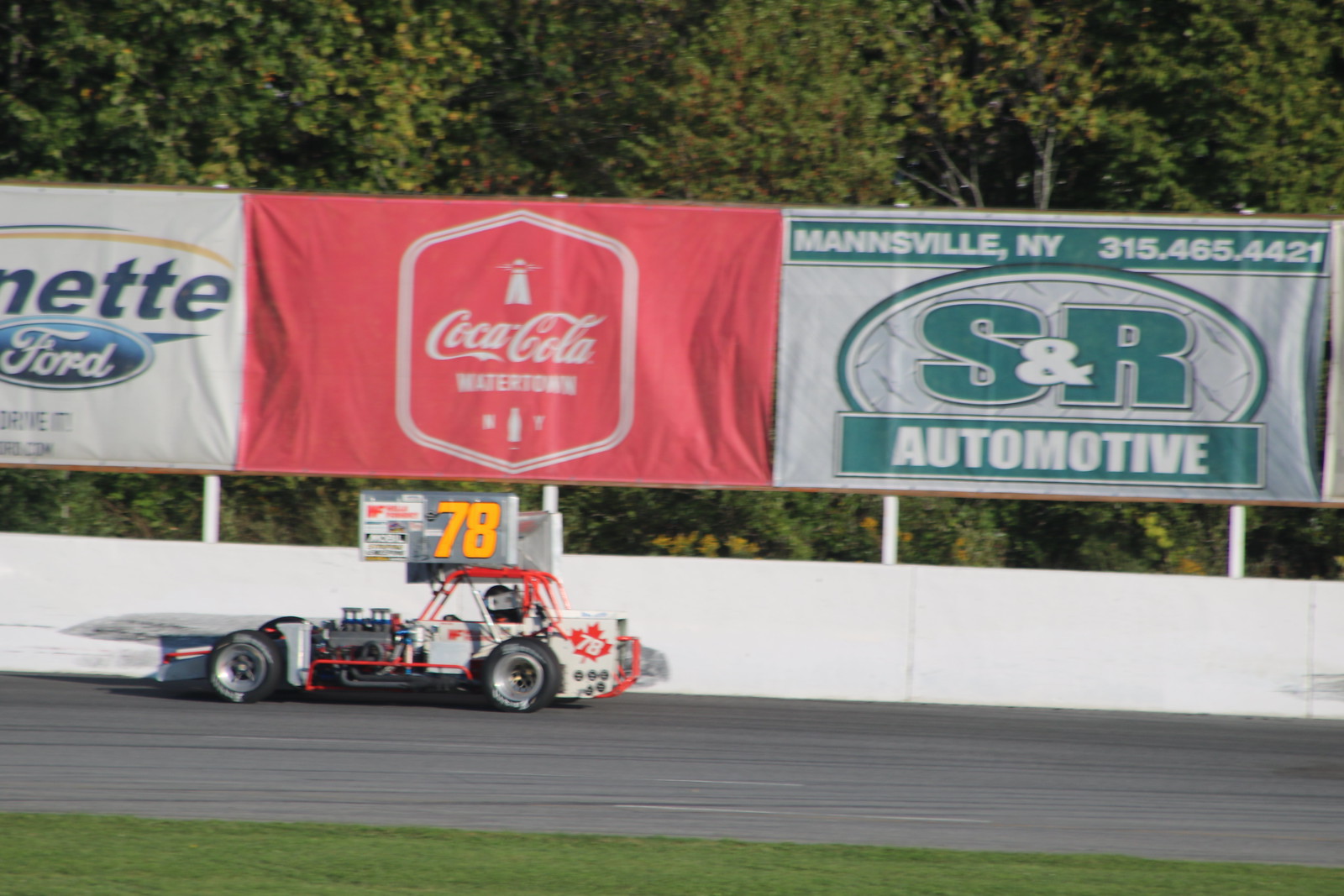In this daytime action shot at an amateur racetrack, a sprint car, decked out in white with red trim and sporting the number 78, zips along the asphalt track with a grassy infield in the foreground. The sleek car is characterized by its aerodynamic features, including a prominent upper wing, a silver engine, bottom wheels, and a red cage protecting the helmeted driver. Above the white boundary wall of the track, several sponsorship banners are visible: a partially cut-off Ford ad on the left, a Coca-Cola ad in the center, and an S&R Automotive ad from Mansville, New York, complete with a phone number. The backdrop extends into a lush environment of green trees and shrubbery, situating the racing action within a natural setting. The car also flaunts a Canadian leaf emblem on the back left corner and numerous other smaller advertisements, which add to its spirited and competitive appearance.